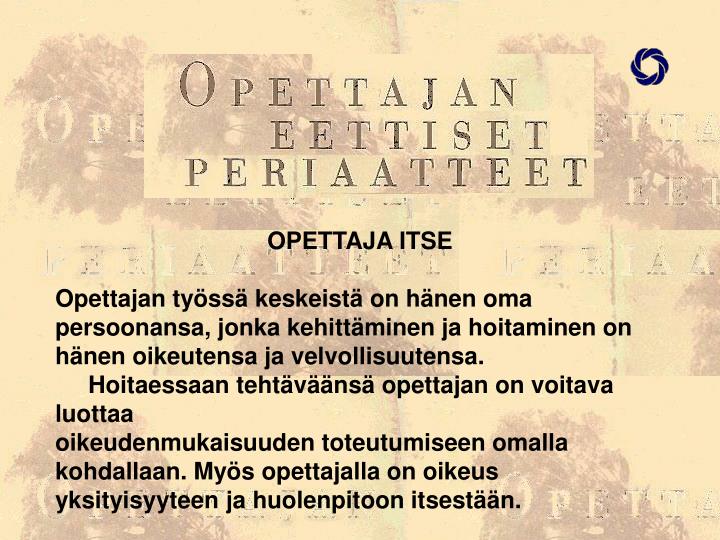The image depicts a rectangular piece of paper with a pinkish beige hue, featuring a PowerPoint slide or poster in a language that is not English. At the top, a centered title in all caps black letters reads: "OPETTAJAN, ETISET, PERIATET." Beneath this, a bold subtitle reads: "OPETAJAITSE." The main body of text, aligned to the left, consists of approximately eight to ten lines, continuing the non-English script in black text. The background of the page gives an impression of an old, historical document, faintly adorned with images of trees situated on the upper left, upper right, middle, and lower corners. The overall background seems to contain faint text or prints, adding to its aged appearance.